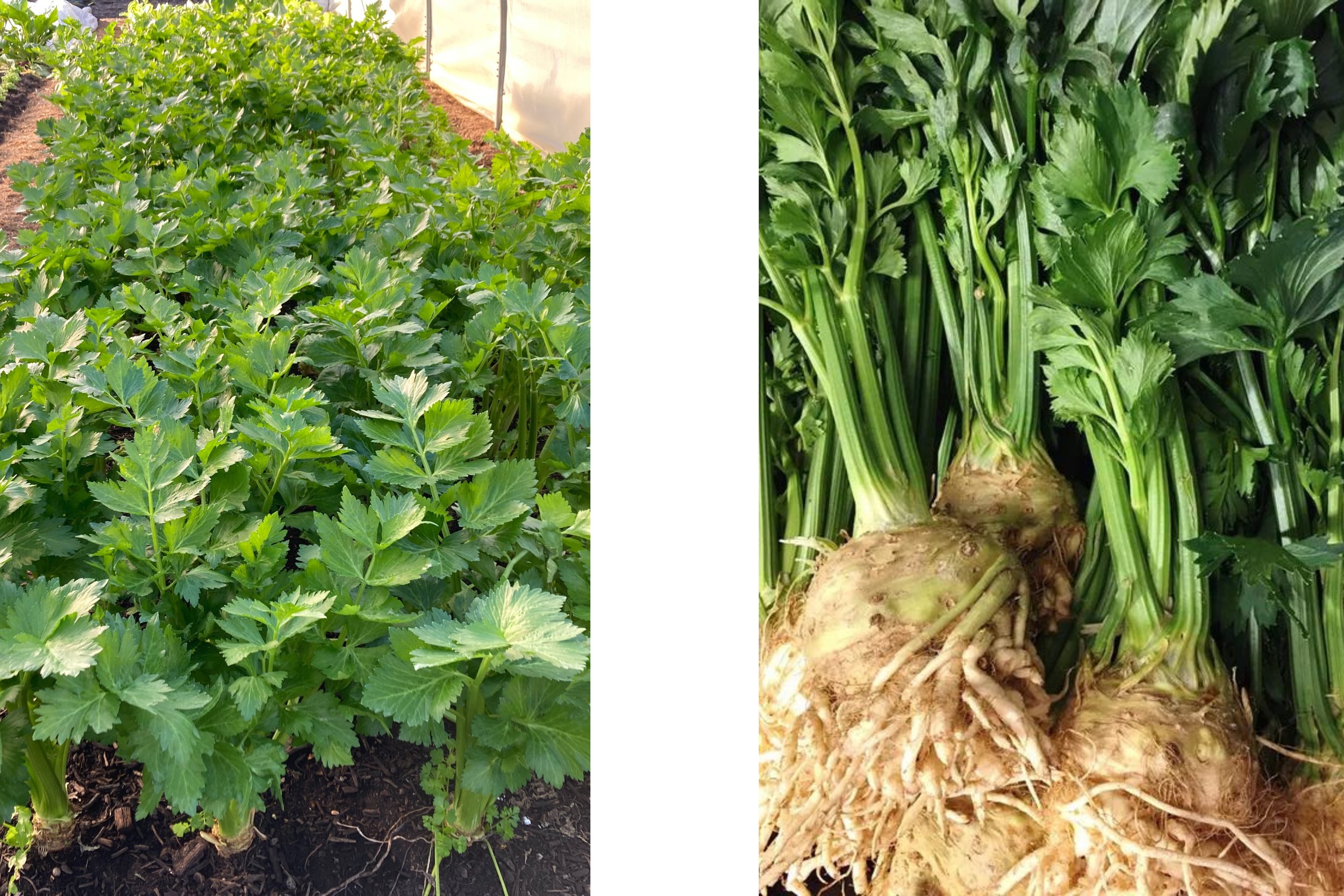The two photographs depict different stages of a celery plant. The left image captures a large vegetable garden where the celery plants are densely grown, appearing almost as a single mass of greenery with their lush, leafy tops. The soil is visible between the scattered and intertwined plants. In contrast, the right photograph focuses on the harvested celery roots, which are large, tannish-brown, and intricately detailed. Some roots form a bell-shaped base before becoming more tube-like and sporadic, with hair-like structures present. The green stalks of the celery are tall, thick, and crowned with fluffy, verdant leaves.